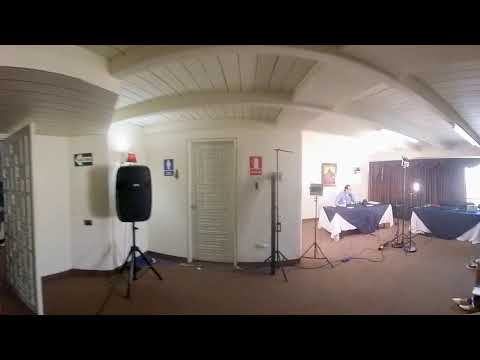The image depicts the inside of a well-lit, white-walled room with a brown carpeted floor and a slatted white wooden ceiling. The focal point is a man, likely Caucasian and wearing a blue button-up shirt, sitting behind a table draped with a white tablecloth and a smaller blue overlay. He appears to be operating a computer or some kind of electronic device. Several spotlights are directed at him, suggesting this could be a press conference or recording session.

In the background, a large red curtain covers windows, with a gap letting in intense sunlight. There are numerous wires and audio equipment scattered around, including what appears to be a speaker on a tripod near the camera. 

To the left, an open door marked with a left-pointing arrow likely indicates an exit, while to the right, near the front, another door adjacent to a men's restroom sign is visible. The room contains multiple tables, including another white and blue-clothed table, reinforcing the setting's organized yet technical atmosphere.